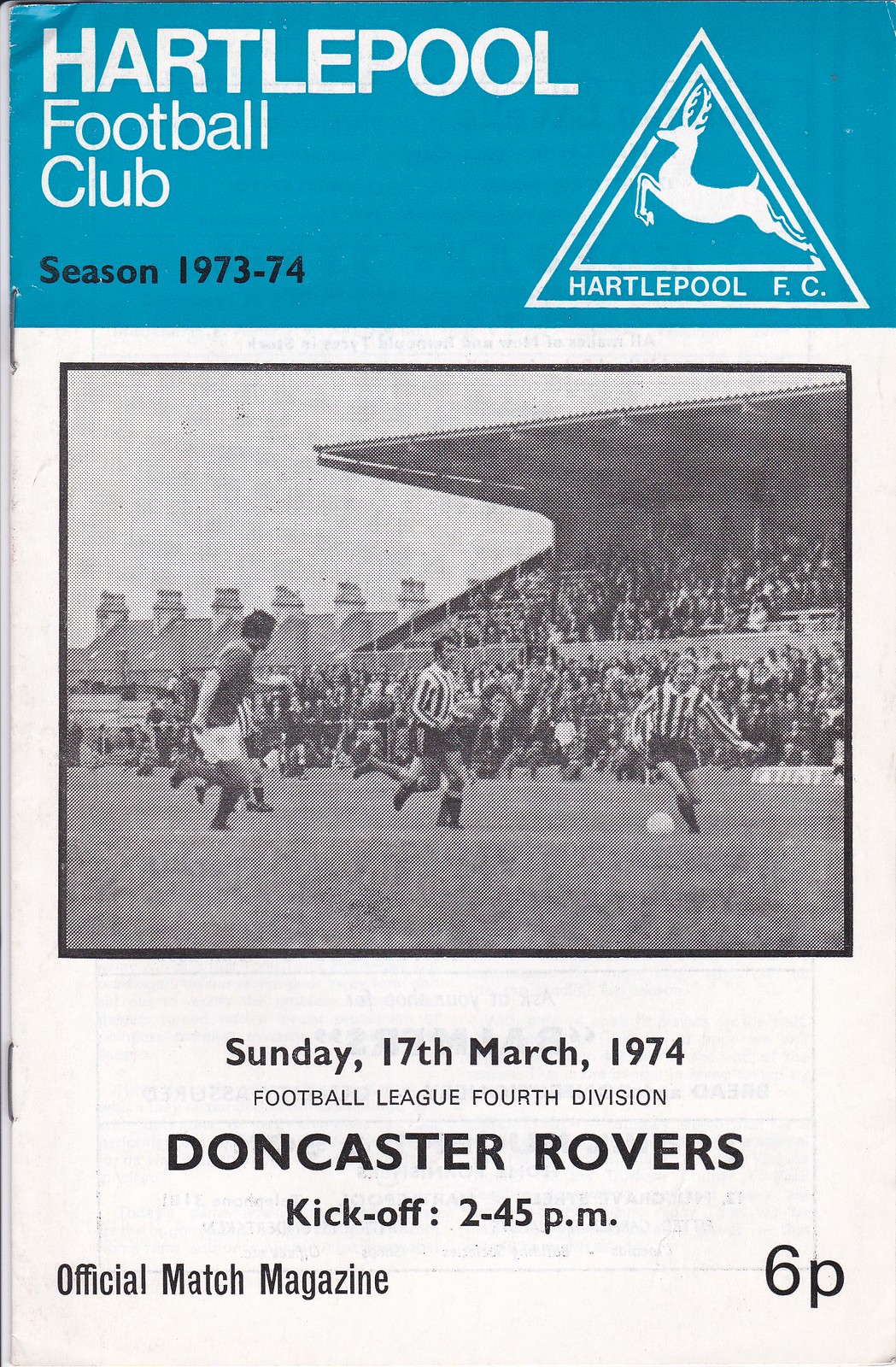This image is of an old sports matchbook program cover for Hartlepool Football Club. The top part of the poster features a blue horizontal strip with white text that reads, "Hartlepool Football Club, Season 1973-1974." On the right side of this strip is a triangular logo featuring a white leaping deer and the text "Hartlepool FC" at the bottom. Below this, centrally located, is a rectangular black and white photograph depicting a soccer match in progress, with players wearing vertically striped jerseys. The photo captures a lively scene with full bleachers and a crowd in the background. The lower portion of the poster, set against a white background, contains detailed event information in black text: "Sunday, March 17, 1974, Football League, 4th Division, Doncaster Rovers, Kick-off 2.45 p.m., Official Match Magazine, 6p." This indicates that the program cover costs six pence.